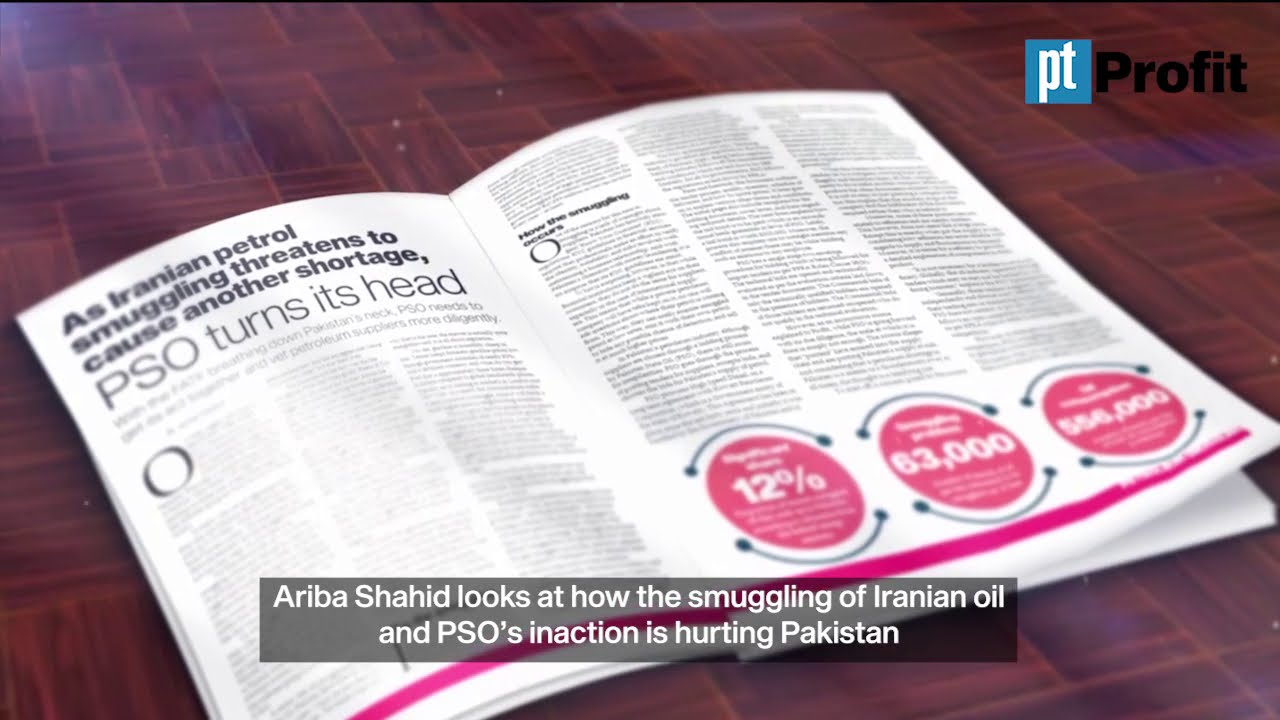The image appears to be an internet advertisement featuring a reddish-brown tiled background. Prominently displayed is an open magazine, lying flat on the floor. In the top right corner of the image, there is a blue box with the logo "PT," and next to it, the black text reads "Profit." The main headline on the left page of the open magazine reads, "As Iranian Petrol Smuggling Threatens to Cause Another Shortage," followed by the subheading "PSO Turns Its Head." The text on the right page of the magazine is mostly unreadable except for three round fuchsia circles, with visible numbers "12%" and "63,000" in the first two circles; the third circle's contents cannot be deciphered. A gray banner at the front of the magazine states, "Ariba Shaheed looks at how the smuggling of Iranian oil and PSO’s interaction is hurting Pakistan." The overall style hints at a possible screenshot from a YouTube video, characterized by its prominent color scheme consisting of red, white, brown, blue, and black.